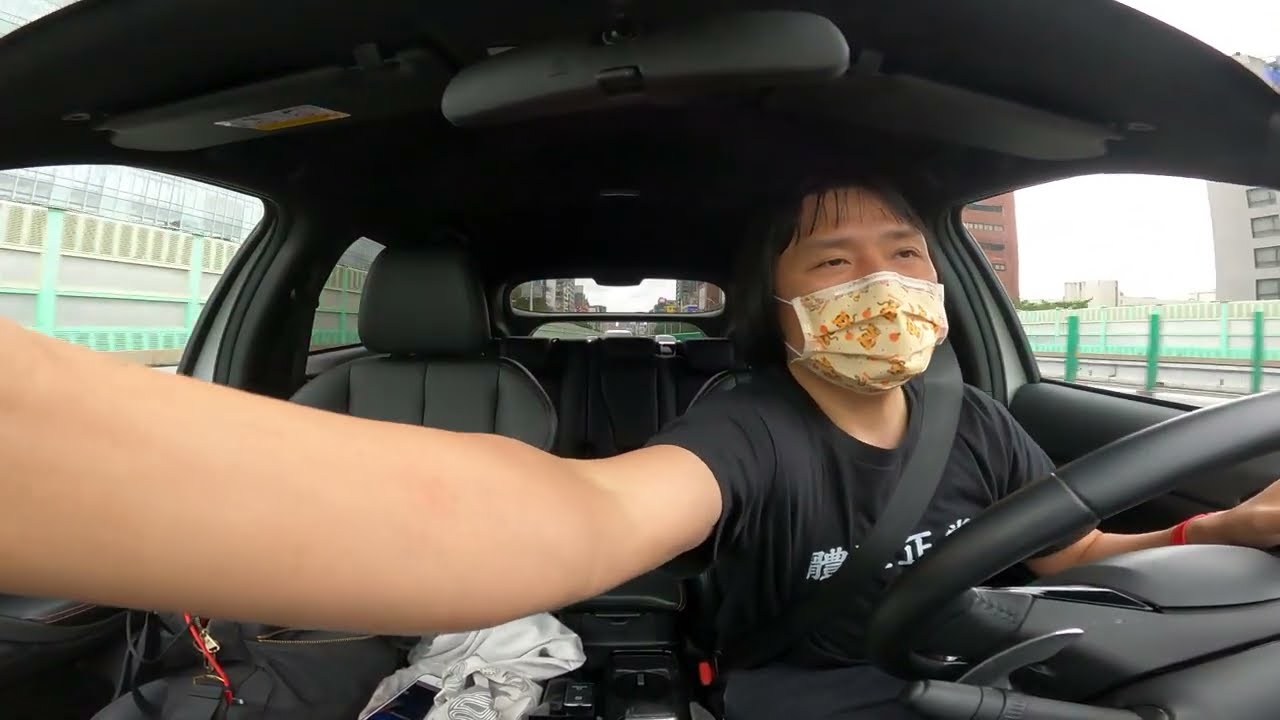In this horizontally aligned, wide rectangular image, we see a person driving a car from the perspective of looking into the front seat. The individual, likely a woman given the visible shoulder-length black hair and bangs, has light brown skin and is wearing a short-sleeve black t-shirt adorned with white symbols in a non-English language. A distinctive orange and yellow patterned mask covers her nose and mouth. Her left hand grips the steering wheel, where a red watch or bracelet can be glimpsed on her wrist, while her right arm appears unusually extended across the frame, creating an illusion of excessive length as it disappears off to the left side of the image. 

Inside the glossy black-leather interior of the car, an empty seat is visible beside her, with a possible white purse or bag resting on it. The rearview mirror is positioned at the top of the image, indicating the photo was taken from the front of the car. Through the windows, we can observe a cityscape with buildings and barriers or fences, suggesting the setting might be an interstate or a busy urban road.